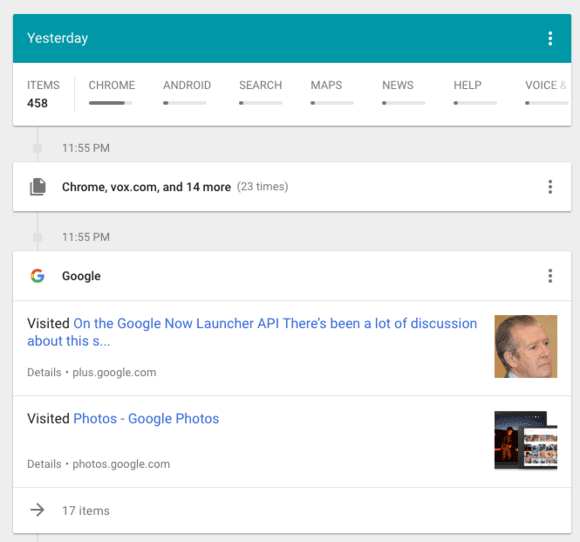This image is a cropped screenshot of the browser history page on a mobile phone. At the top, there is a green banner displaying the word "Yesterday" in large white letters on the left side. To the right, three vertically aligned dots are visible, likely representing a menu icon.

Below the green banner, there is a white box. On the far left side of this box, the text "Items 458" is displayed. To the right, there is a vertical list of categories, each accompanied by a small gray progress bar. 

- The first category is "Chrome," which has a nearly full progress bar.
- "Android" follows, with only a small portion of the left side of the bar filled.
- "Search" also shows minimal progress.
- "Maps," "News," "Help," and "Voice" categories each have no progress indicated.

Further down, the screenshot displays the timestamp "11:55 PM" in small gray font. Below this timestamp, there is another white box. At the top left of this box, it says "Chrome," followed by "vox.com and 14 more," with "23 times" indicated in small gray font within parentheses. 

At the very bottom, the timestamp "11:55 PM" is shown again in small gray font. Below this, there is a larger white box with "Google" at the top left corner, which likely lists various websites visited by the user at that time, each entry accompanied by the same timestamp of "11:55 PM."